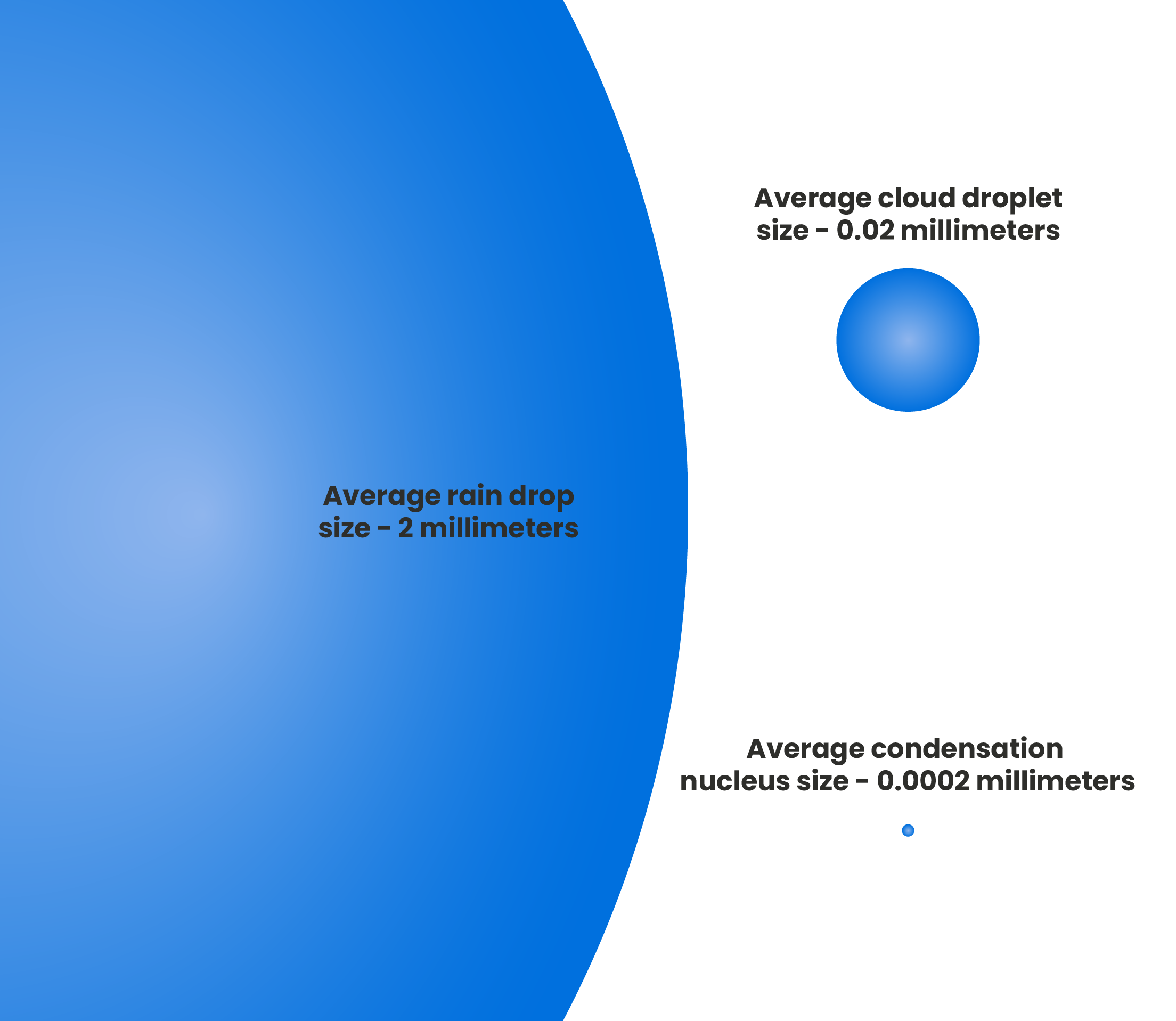The image features a comparison of different droplet sizes, presented on a contrasting blue and white background. On the left side, a large blue area contains a text label that reads "Average raindrop size - 2 millimeters." On the right side, a white background showcases a blue circle with the text "Average cloud droplet size - 0.02 millimeters" above it. Below this blue circle, at the very bottom of the image, a minuscule blue dot is visible, accompanied by the text "Average condensation nucleus size - 0.0002 millimeters." The image effectively illustrates the vast differences in size between raindrops, cloud droplets, and condensation nuclei.